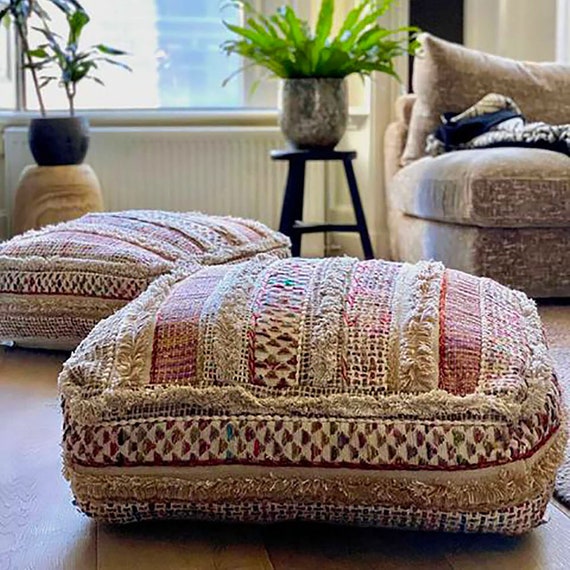This is an indoor photograph of what appears to be a cozy living room scene. The focal point is two large, plush throw pillows with vibrant colors and intricate patterns, lying on a brown hardwood floor. The pillow in the foreground is multicolored, featuring strips of beige and white, covered with a multitude of multicolored triangles and other designs in red and white. Another pillow, similar in style, lies slightly behind and to the left. 

In the background, a window allows natural light to enter, illuminating a variety of elements. Beneath the window is a beige wall, and in front of it stands a white furnace. To the left of the furnace, there's a black barstool topped with a marbled vase containing a lush green plant. Further to the left and on a tan stool, there's another plant in a black pot with tall, grassy foliage.

On the right side of the image, the edge of a beige couch can be seen, covered partially with a blue blanket. The overall scene is filled with warm, earthy tones and a mix of textures, creating a welcoming and comfortable atmosphere.